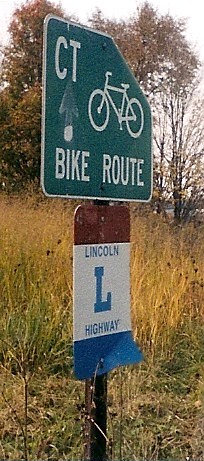In this photograph taken near a street, we see a notable signpost positioned against a backdrop of dry, tall grass and sparse autumn trees. The image prominently features two signs mounted on the post. The top sign is square and green with white capital letters "CT" in the upper left corner, accompanied by an upward-pointing arrow, although the arrow’s paint is somewhat chipped. Below the arrow, the words "BIKE ROUTE" are displayed in white, with a white bicycle symbol above the word "ROUTE." The lower sign is vertically rectangular with three colored sections: red at the top, white in the middle, and blue at the bottom. Within these sections, the words "LINCOLN HIGHWAY" are written in blue, with "LINCOLN" in the white section and "HIGHWAY" in the blue section, separated by a large blue "L." This detailed scene captures the essence of an outdoor pathway, complete with street signage and a serene, dry autumn landscape.